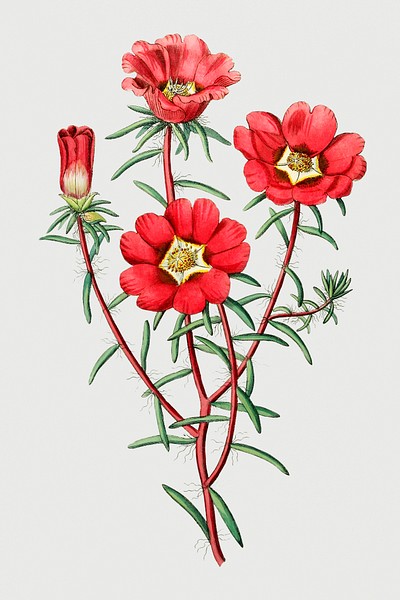This vertical rectangular image showcases a vibrant digital artwork of four blooming flowers attached to their stems. The flowers, painted in a rich red with sunny yellow centers, stand out vividly against a crisp white background. Each flower has lush green leaves sprouting from its base, enhancing the natural beauty of the composition. These green leaves are scattered along red stems, which also display tiny hair-like structures near the points where the leaves attach, adding texture and realism. The arrangement of the flowers is eye-catching: two are positioned at the center, one above the other, while the remaining two are placed to the left and right, respectively. Notably, the flower on the left is currently closed, adding an element of anticipation. The overall effect is a harmonious blend of colors and details that make the artwork come to life.